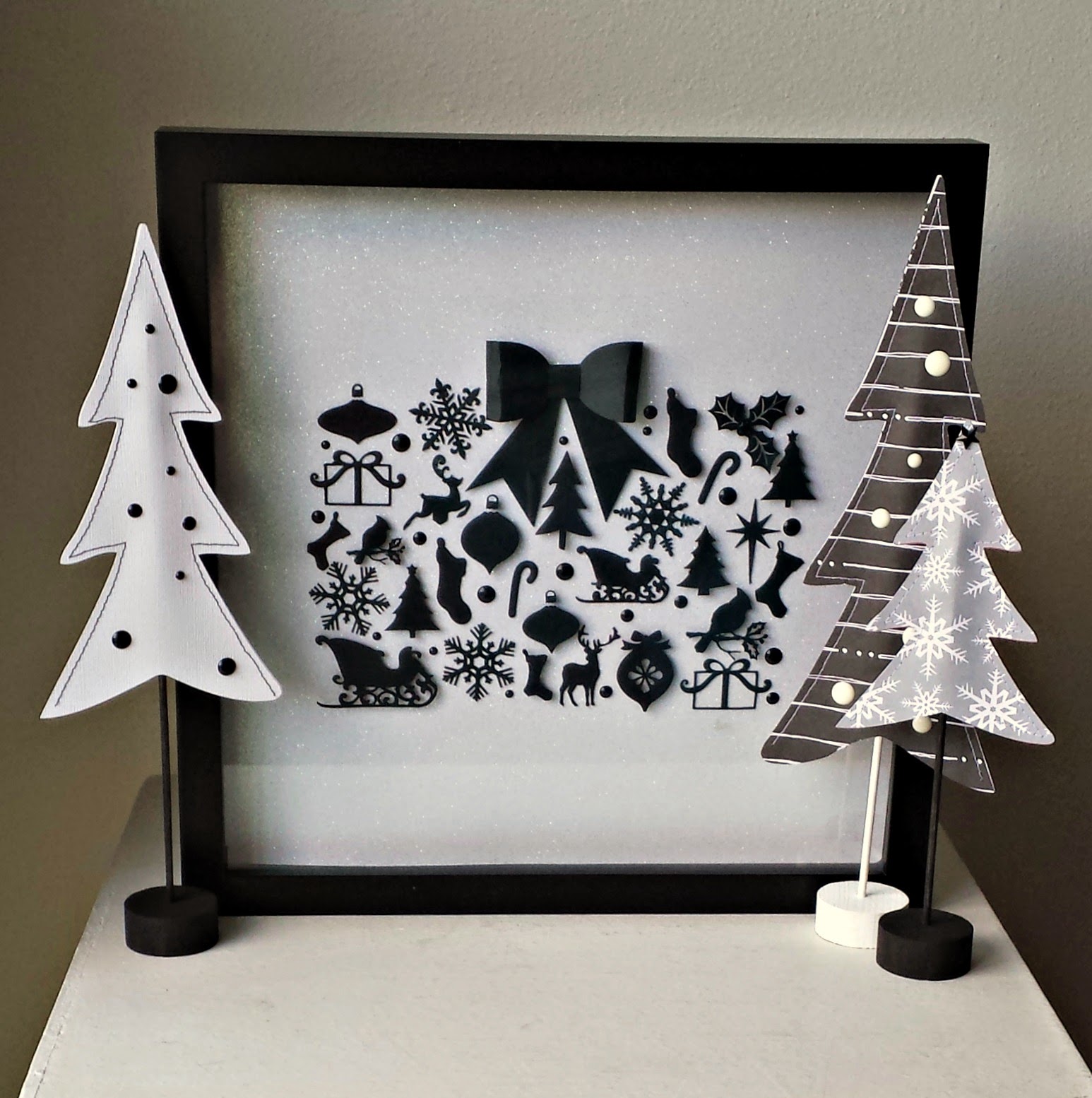This photograph features a detailed arrangement of black and white Christmas decorations. At the center is a square black picture frame set against a gray background, showcasing a variety of intricately cut black silhouettes of festive icons. These include reindeer in mid-jump, Santa's sleigh, stockings, Christmas trees, candy canes, wrapped presents with bows, sprigs of holly, snowflakes, a cardinal bird on a branch, and assorted ornaments. These symbols repeat several times within the frame.

Flanking the frame are three small, cloth Christmas trees on slender stands, adding dimension to the display. The trees are black, white, and black-and-white in color, positioned on top of round black or white puck-shaped bases. All of these elements rest on a square, white side table, set against a gray wall, creating a minimalist yet festive scene. The photograph appears to be taken indoors from a straight-on angle, capturing the monochromatic decor with a clear emphasis on the framed Christmas icons as the focal point. The overall color palette includes shades of black, white, gray, and off-white, contributing to the crisp and elegant atmosphere of the display.